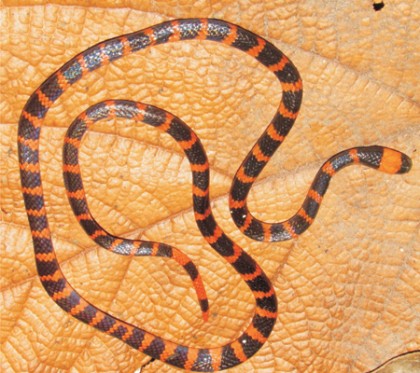This photograph features a small, vividly-striped snake with alternating black and orange bands along its slender body. The snake's head, which is positioned towards the middle-right side of the image, is black, and the striping pattern continues consistently down to its orange-tipped tail. The snake is laid out in a relaxed, slightly coiled manner, resembling a loose spaghetti noodle rather than a tightly wound coil. It rests atop a large, muted orange leaf with prominent veining, which suggests a leathery texture. The close-up perspective of the image highlights both the intricate details of the snake's pattern and the textured surface of the leaf, creating a lifelike and detailed depiction.